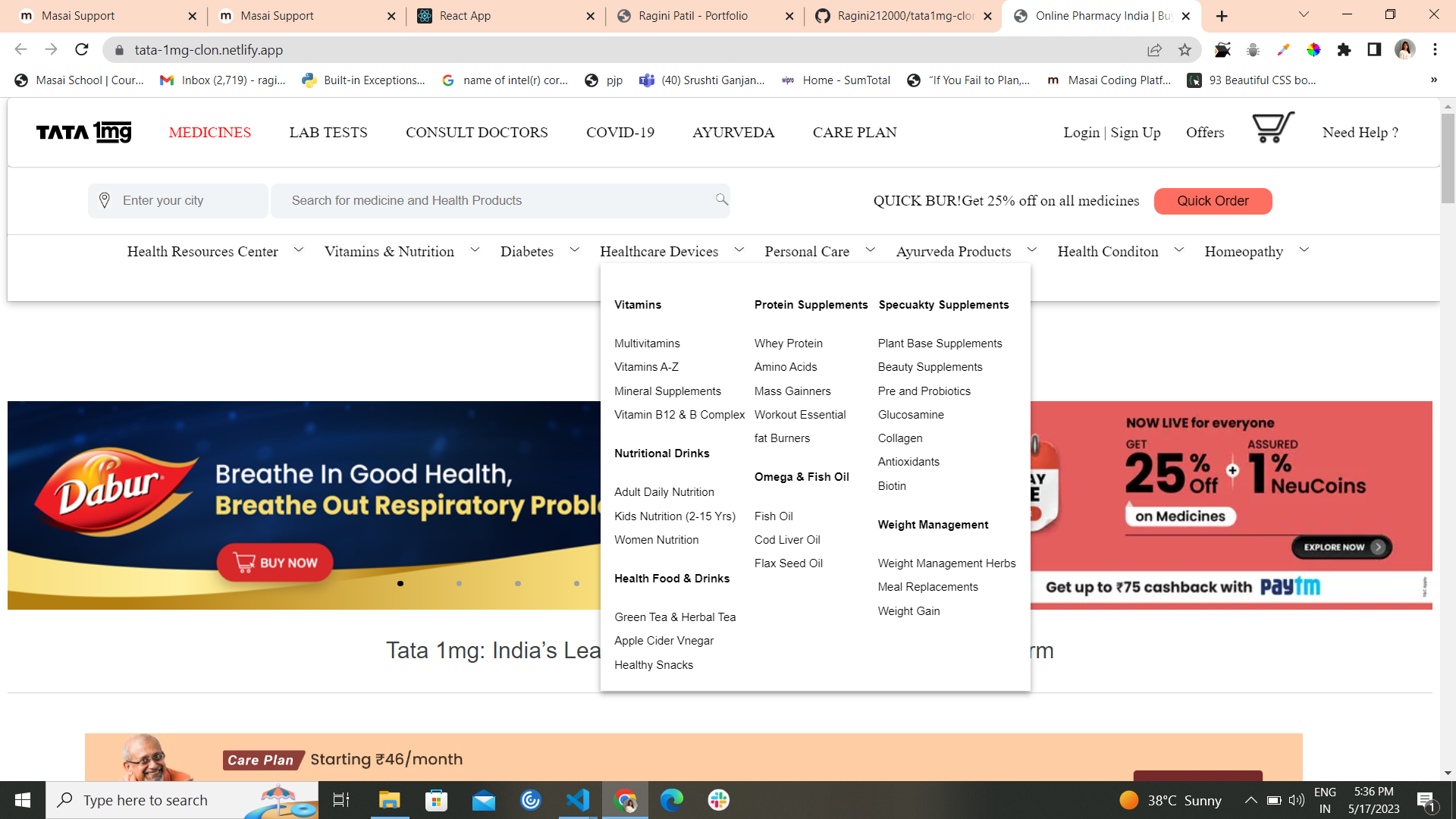**Descriptive Caption:**

The image depicts the homepage of the Tata 1MG online pharmacy platform as displayed in a React application. The main color scheme of the interface is pink, which signifies the user-selected theme. The address bar shows the URL "tata-1mg.netlify.app". 

At the top of the screen, the site’s header includes navigation options such as "Medicines", "Lab Tests", "Consult Doctors", "COVID-19", "Ayurveda", "Login", "Sign Up", and "Offers". Below the header, there is an extensive search bar where users can search for medicines and health products, with a highlighted quick order option offering a 20% discount on all medicines.

The site provides a detailed categorization of products spanning various health needs:
- Vitamins and Supplements (including multivitamins, vitamin A to Z, vitamin B12, and B-complex)
- Protein Supplements (such as whey protein, amino acids, and mass gainers)
- Workout and preparation aids
- Plant-based supplements and probiotics
- Health products like glucose, collagen, and omega fish oil
- General nutrition for adults and kids
- Health foods and drinks, such as green tea, herbal tea, and apple cider vinegar
- Weight management staples

Additionally, the site features sections dedicated to health resources, focusing on building good health and managing respiratory problems, with a "Buy Now" prompt offering a 20% discount for new clients. The Tata 1MG Microsoft symbol is positioned at the bottom-left of the screen, completing the page design.